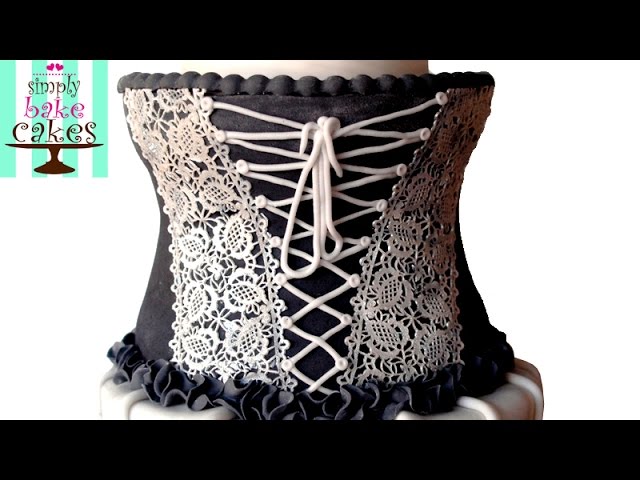This landscape-oriented color photograph features a highly detailed cake designed to resemble a woman's chest adorned with a black lace bustier. The cake showcases intricate craftsmanship with its concave sides and a V-shaped front, tied together with elegant white lace strings. Black scallops decorate the top and bottom edges of the bustier, adding to its realistic appearance. The cake is displayed on a white cake stand.

In the upper left corner of the image, there is a poster for Simply Bake Cakes. The logo is set against a backdrop of diagonal light green and white stripes. It features a brown cake stand topped with two pink hearts, followed by the text "Simply" in a dark-colored font, "Bake" in a light pink font, and "Cakes" in a brown font, all in ornate script. The image is framed with horizontal black stripes at the top and bottom, and the background is primarily white, emphasizing the photographic realism of the cake.